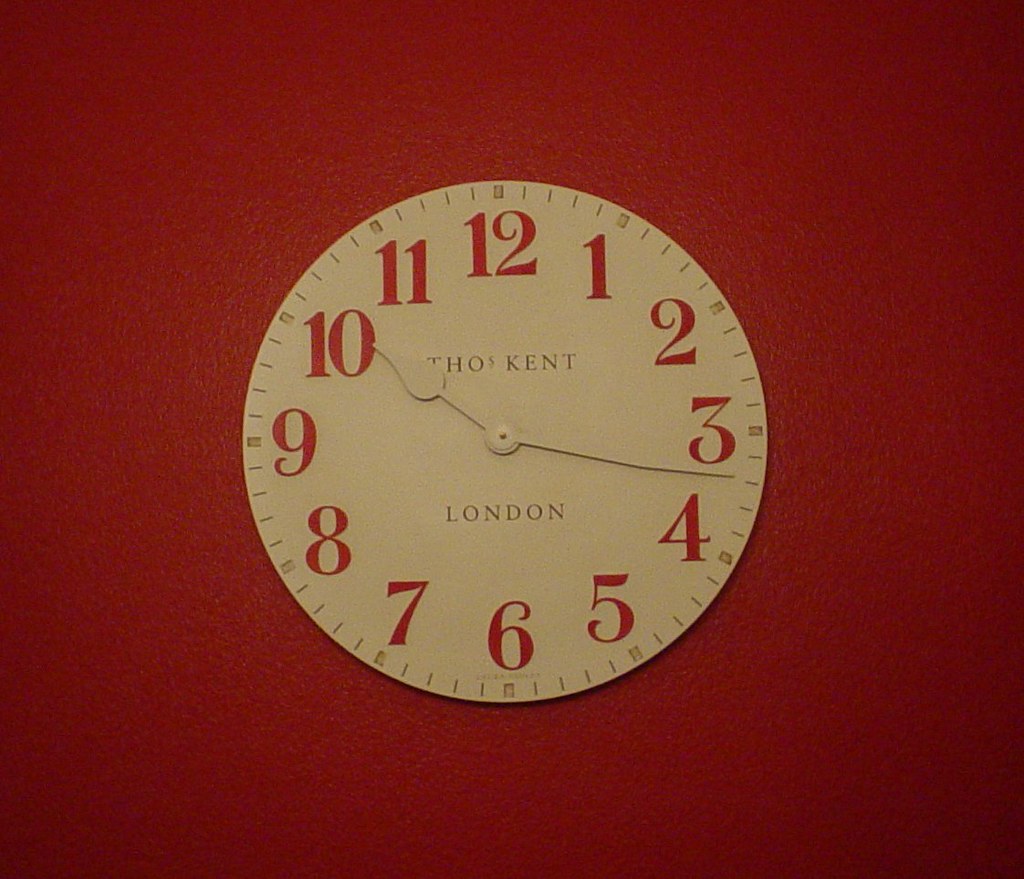This photograph captures a minimalist white clock face mounted on a richly painted red wall. The clock, appearing to be made of either plastic or paper, lacks any visible frame or mounting structure, emphasizing its simplicity. The dial prominently features large red numbers from 1 to 12 and sleek black minute hatch marks, with thicker, block-like markings at each five-minute interval. The clock shows the time as 10:17, with a large, teardrop-shaped hour hand pointing near the 10 and a substantial minute hand at 17. Above the center of the dial, the inscription "THOS Kent" is visible, and below that, it reads "London." The second hand is straight, contributing to the straightforward elegance of the timepiece.